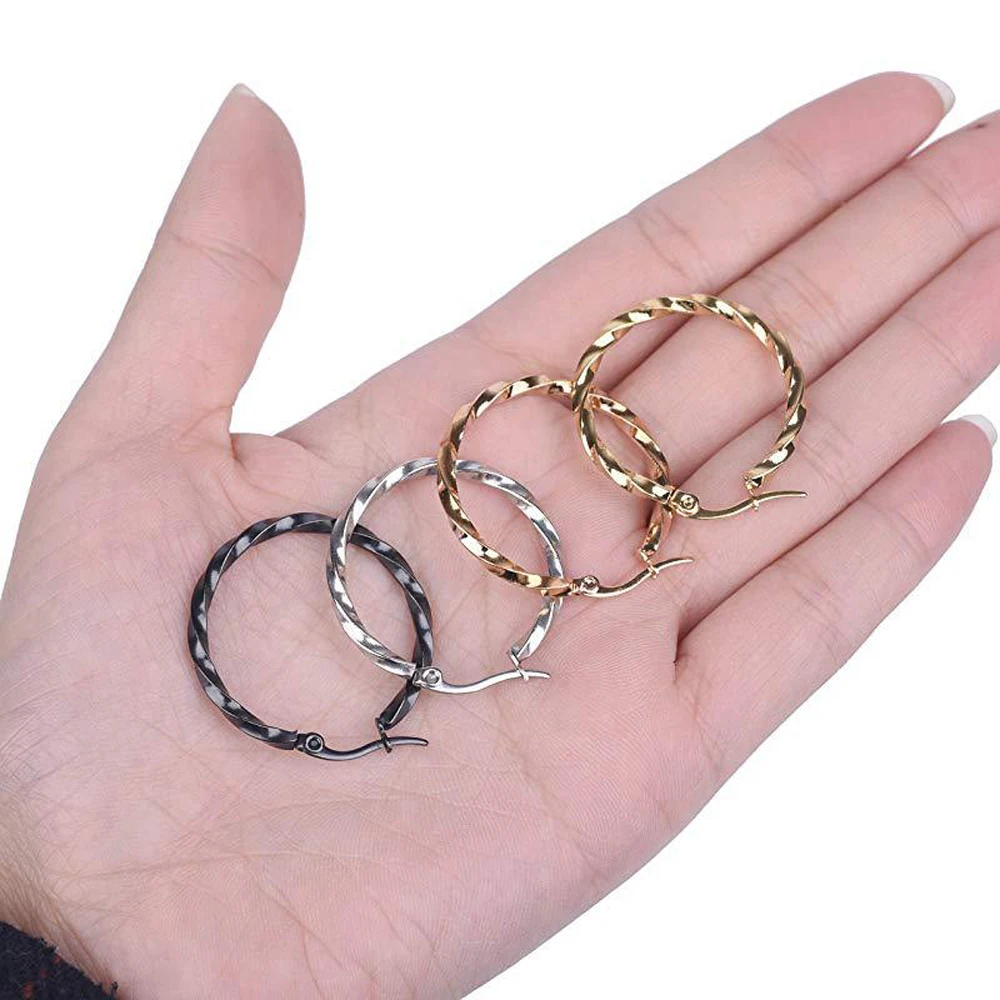In this bright, rectangular, horizontally-aligned photograph, we see a diagonally-oriented, possibly feminine, left hand with long, sculpted, rounded fingernails. The hand, appearing young and Caucasian, is palm-up with fingers aligned closely together and the thumb pointing upwards to the right, creating a small gap. At the center of the palm, four hoop earrings rest in an accordion-like fashion, layered predominantly from left to right and slightly overlapping. The leftmost earring is a darker grey, followed by a lighter silver one, then a rose-gold colored hoop, and finally, a yellow gold hoop. These almost perfect circular earrings are either twisted metal or painted plastic, each featuring a slightly curved stake and screw attachment for piercing. The white background is stark and clear, enhancing the focus on the hand and earrings, suggesting this could be an advertisement for the jewelry. Black material, possibly part of the wrist area, is slightly visible.